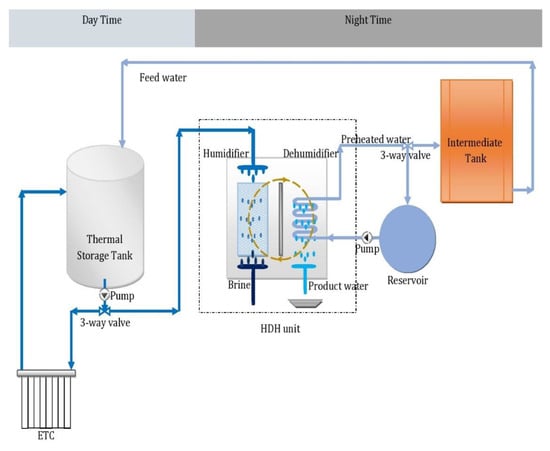The image depicts a detailed flowchart against a mostly white background, illustrating a thermal storage and water processing system. At the top of the chart, two bars are displayed: a lighter gray bar labeled "daytime" and a larger, darker gray bar labeled "nighttime." Below, a labeled cylinder representing the "thermal storage tank" is central, with blue arrows indicating the flow of materials. Connected to the thermal storage tank are a "pump" and a "three-way valve." From this valve, pathways lead to a "humidifier," and then to a "dehumidifier." The humidifier, depicted like a shower head, combines with brine before reaching the dehumidifier, which then generates both "product water" and "preheated water." The preheated water either returns to the three-way valve, linking back to the reservoir and pump in a continuous loop, or goes to an "intermediate tank." This intermediate tank then initiates a "feed water" process, refeeding into the thermal storage tank, indicating a cyclical system. Additional elements of the system include an "HCH unit" and various flow connections, suggesting a complex air handling and water circulation HVAC system.